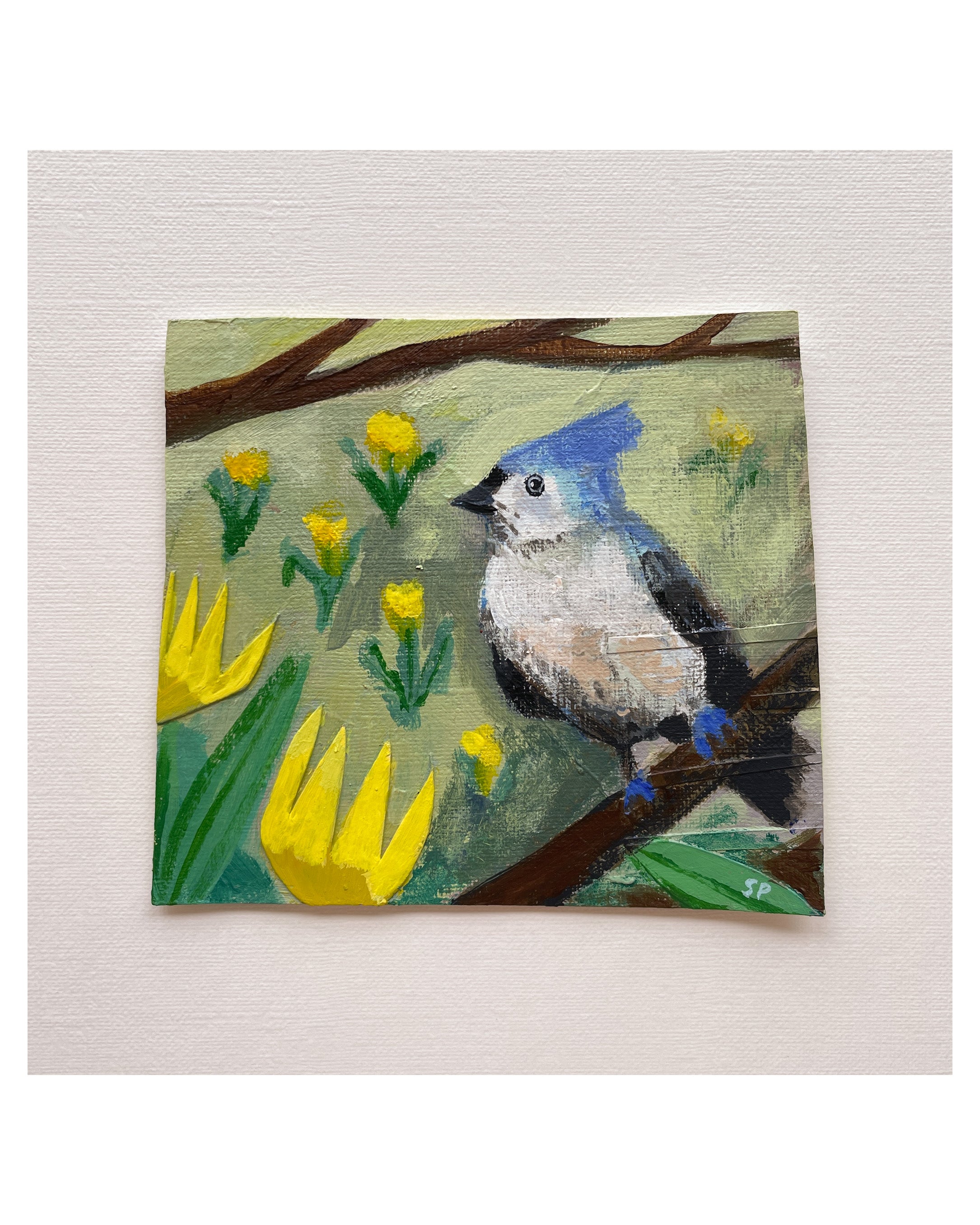This is a photograph of a painting centered on what appears to be a plain white fabric canvas. The painting depicts a vibrant blue and white bird, likely a blue jay, perched on a brown stick adorned with a single green leaf. To the left of the bird are several yellow flowers, possibly resembling daffodils or daisies, accompanied by striking green leaves. An additional brown stick at the top of the painting frames the composition. In the bottom right corner, the initials "SP" are inscribed in small white text, presumably the artist's signature. The painting, which appears to be created with acrylic or oil, is small and square in shape, but exact dimensions are not provided.